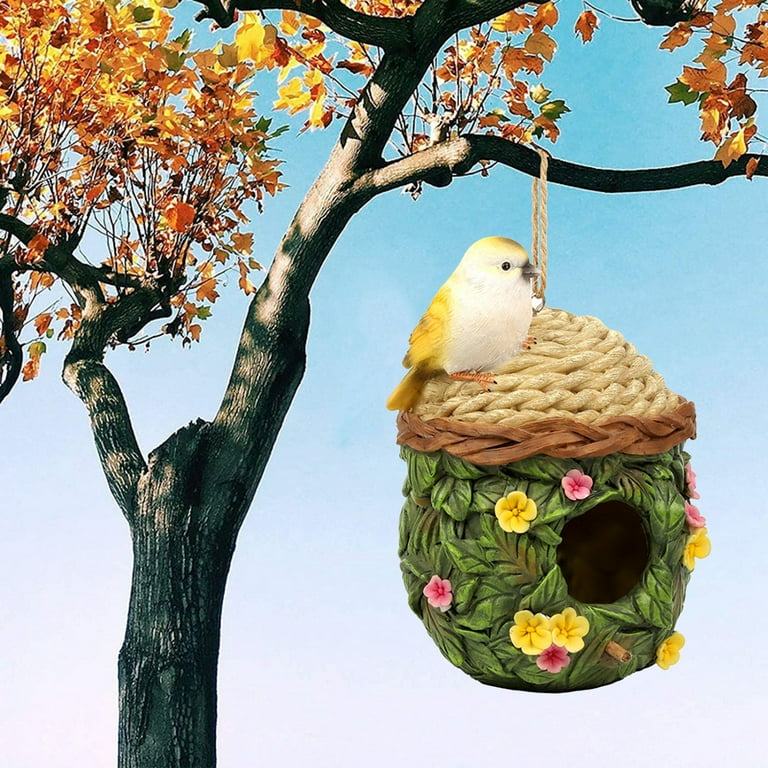This vertical rectangular image depicts a creatively edited photograph featuring a tree adorned with brown and yellow autumn leaves, rich branches extending in various directions, and a picturesque blue sky in the background that gradually transitions to a light blue hue with hints of red. Dominantly suspended from one of the tree's good-sized branches is an unusual, photoshopped birdhouse that stands out with its distinctive design.

The birdhouse is primarily green, akin to ceramic, embellished with artistic carvings of green leaves, and decorated with intricate pink and yellow flowers. Its roof is composed of a wicker-like material made of white and brown rope, giving it a knitted appearance. Attached by a visible gray string or cord, it seems delicately held against the backdrop tree branch.

Perched on the roof of this whimsical birdhouse is a small bird, characterized by a white body accented with a yellow head, yellow wings, and tail, along with bright orange feet, providing a lively contrast to the green of the birdhouse. Despite the compelling realism of the bird, there's a certain artifice, hinting that it might also be digitally added. The central opening of the birdhouse suggests an entrance for the bird, likely equipped with an understated perch that blends subtly into the design.